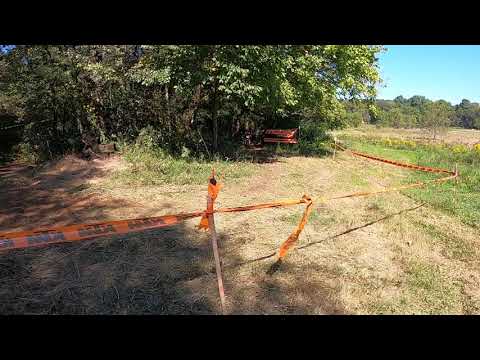The photograph, framed with a black header and footer, captures a scene taken during the daytime in a grassy, park-like outdoor area. The focal point is an orange caution tape, inscribed with unreadable black writing, stretched tautly between small wooden posts or stakes anchored in dry ground, interspersed with patches of green and dead grass. The tape partitions off a section leading towards a dense cluster of tall, green trees, suggesting an area that's off-limits. Behind these trees, there is a heavily forested region under a bright, clear blue sky. Subtly visible within the wooded backdrop is a blurry, rectangular reddish object, possibly the back end of a pickup truck or a sign, hinting at some ongoing activity or an area under preparation, likely preventing vehicular access.